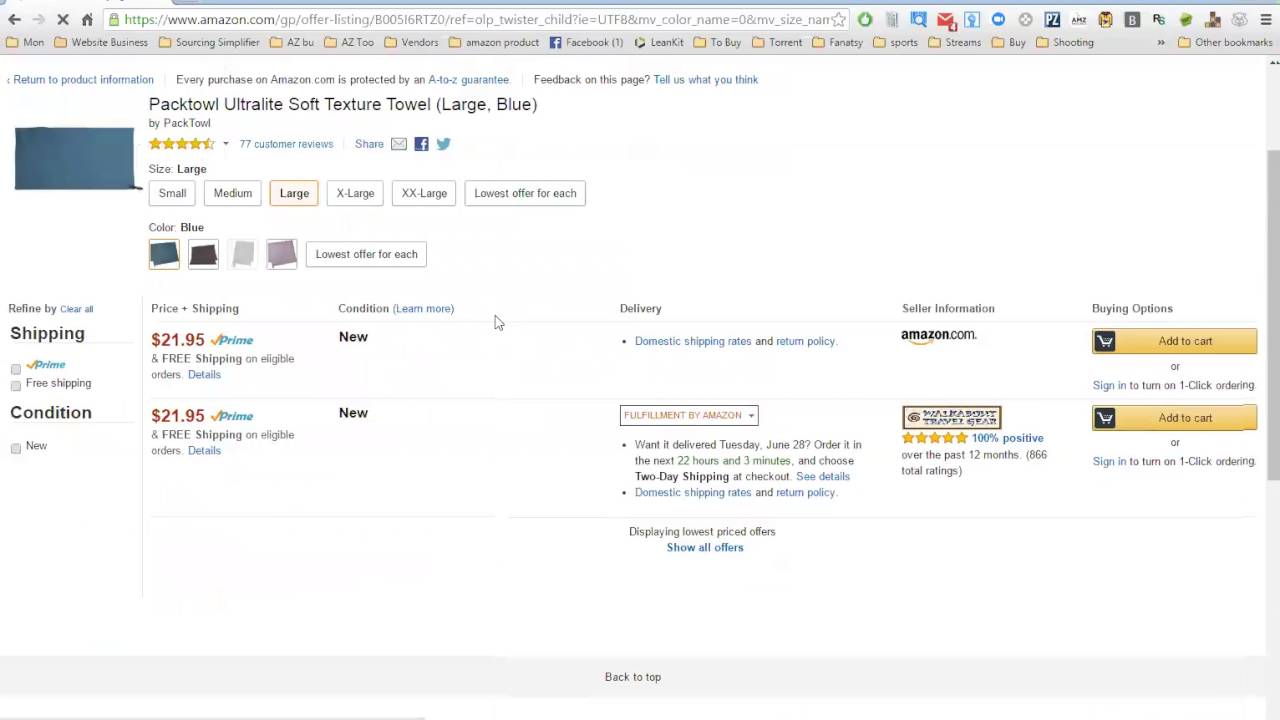The image depicts a web browser window open to Amazon.com with a single tab displaying the product page for the Pactowl Ultralight Soft Texture Towel. This particular listing is for the large blue version of the towel, manufactured by Pactowl. The product boasts an overall rating of 4.5 stars based on 77 customer reviews. Social media sharing options for the product are available via email, Facebook, and Twitter. 

A detailed image of the towel is prominently displayed on the left side of the page. The towel is available in multiple sizes: small, medium, large, extra-large, and extra-extra-large, with pricing and shipping options provided for each size. Additionally, the towel comes in several color choices, including blue, black, white, and pink. 

The price for the large blue towel stands at $21.95 with free shipping on eligible orders, and the product is fulfilled by Amazon, ensuring reliable delivery. Customers can expect their orders to be delivered by Tuesday, June 28th if placed within the next 22 hours and 3 minutes, with the option of selecting two-day shipping at checkout. Links to "Domestic shipping rates" and "Return policy" are accessible and highlighted in blue. The website interface is clear and user-friendly, with a strong emphasis on customer satisfaction, as evidenced by the prominently displayed ratings and reviews.